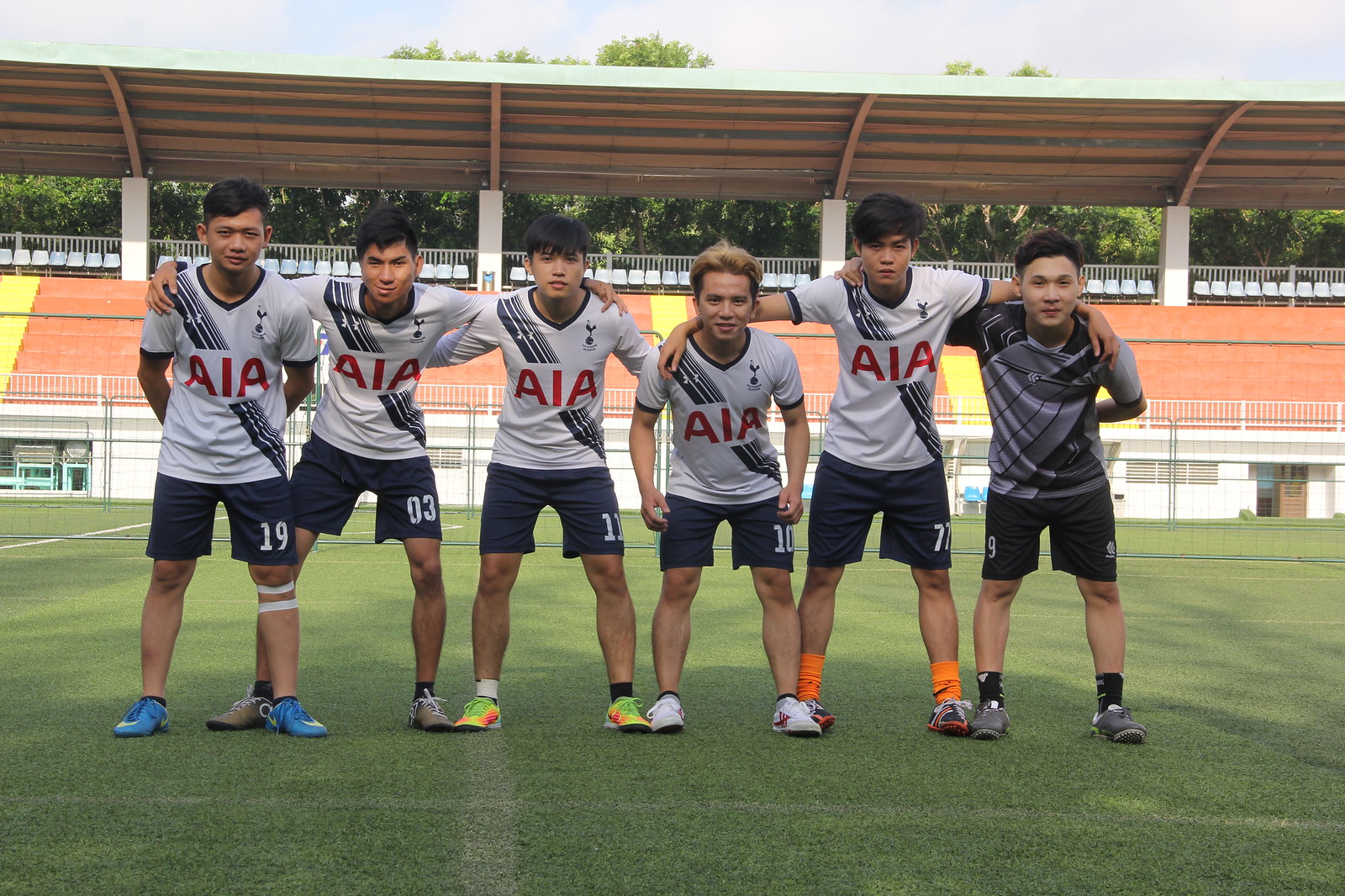The image captures a group of six teenage male soccer players, centrally positioned on a meticulously maintained grass field marked with white lines. They are dressed uniformly in white shirts with black stripes and navy blue or black shorts displaying their team numbers. The shirts prominently feature "AIA" text. Notably, the boy on the far left has two bands around his knee. All players are equipped with cleats and are looking directly towards the camera.

In the background, several rows of seating, including empty orange stands topped with a row of white chairs, can be seen. Above the stands, there is a light green metal awning providing shade. A thin net-like fence is situated behind the players, and the scene is framed by some trees and a sliver of the sky, indicating an outdoor setting on a clear day. The setting appears to be a stadium, possibly during midday, providing a vivid and detailed depiction of a soccer field.